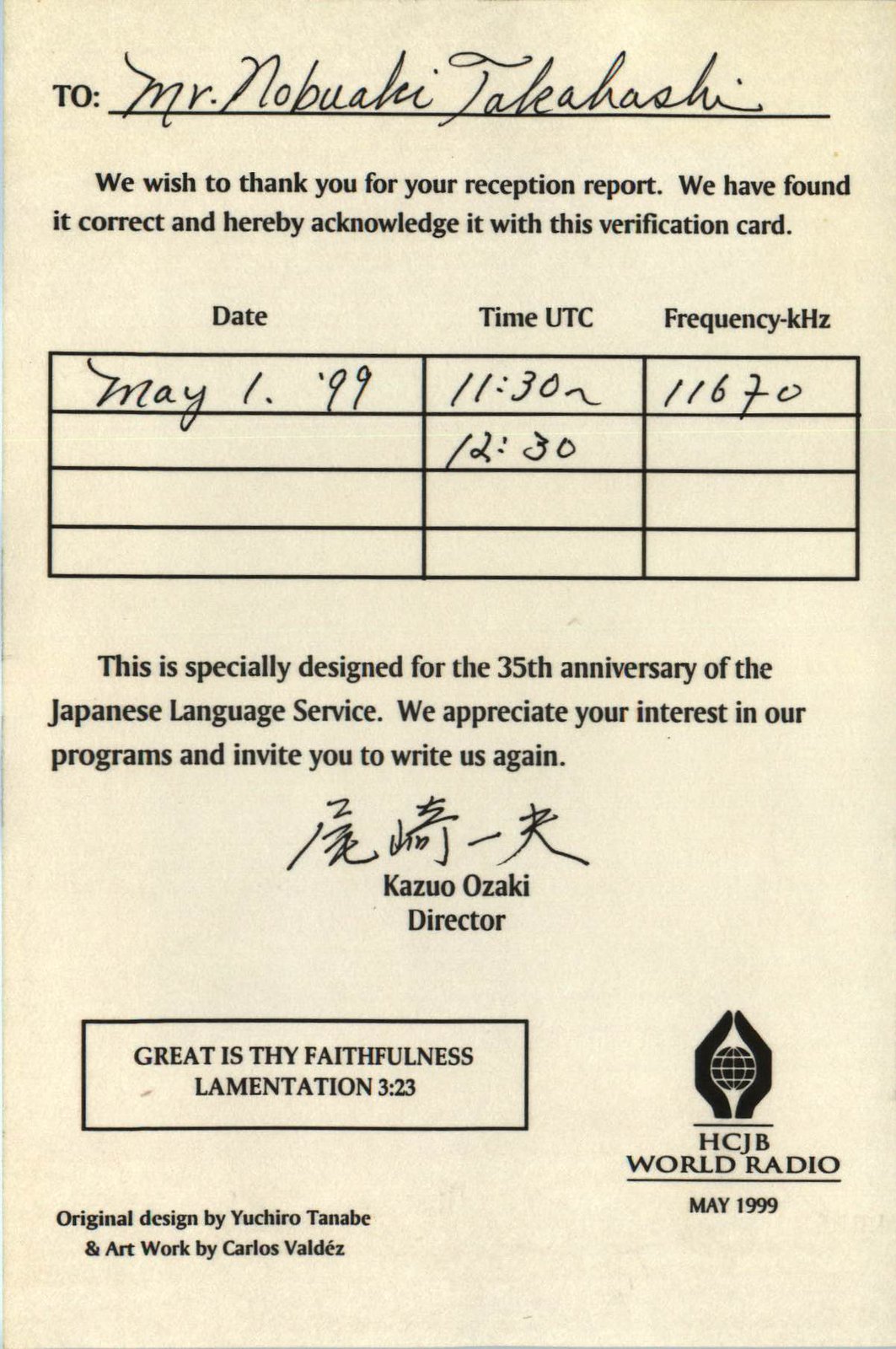The image showcases a detailed verification card from HCJB World Radio, addressed to Mr. Noboki Takahashi. It prominently reads, "We wish to thank you for your reception report; we have found it correct and hereby acknowledge it with this verification card." The card is filled in with specific details: the date is May 1st, 1999, the time is 1130 UTC, and the frequency is 11670 kHz. This card was specially designed for the 35th anniversary of the Japanese Language Service, and it expresses appreciation for the recipient's interest in their programs, inviting further correspondence. The card bears the signature of Kazuo Ozaki, Director, and features the quote, "Great is thy faithfulness," from Lamentations 3:23 at the bottom. The logo of HCJB World Radio is visible on the right, with the design attributed to Yuichiro Tanabe and artwork by Carlos Valdez. The entire image is in black and white, with clean and well-spaced text giving it a postcard-like appearance.